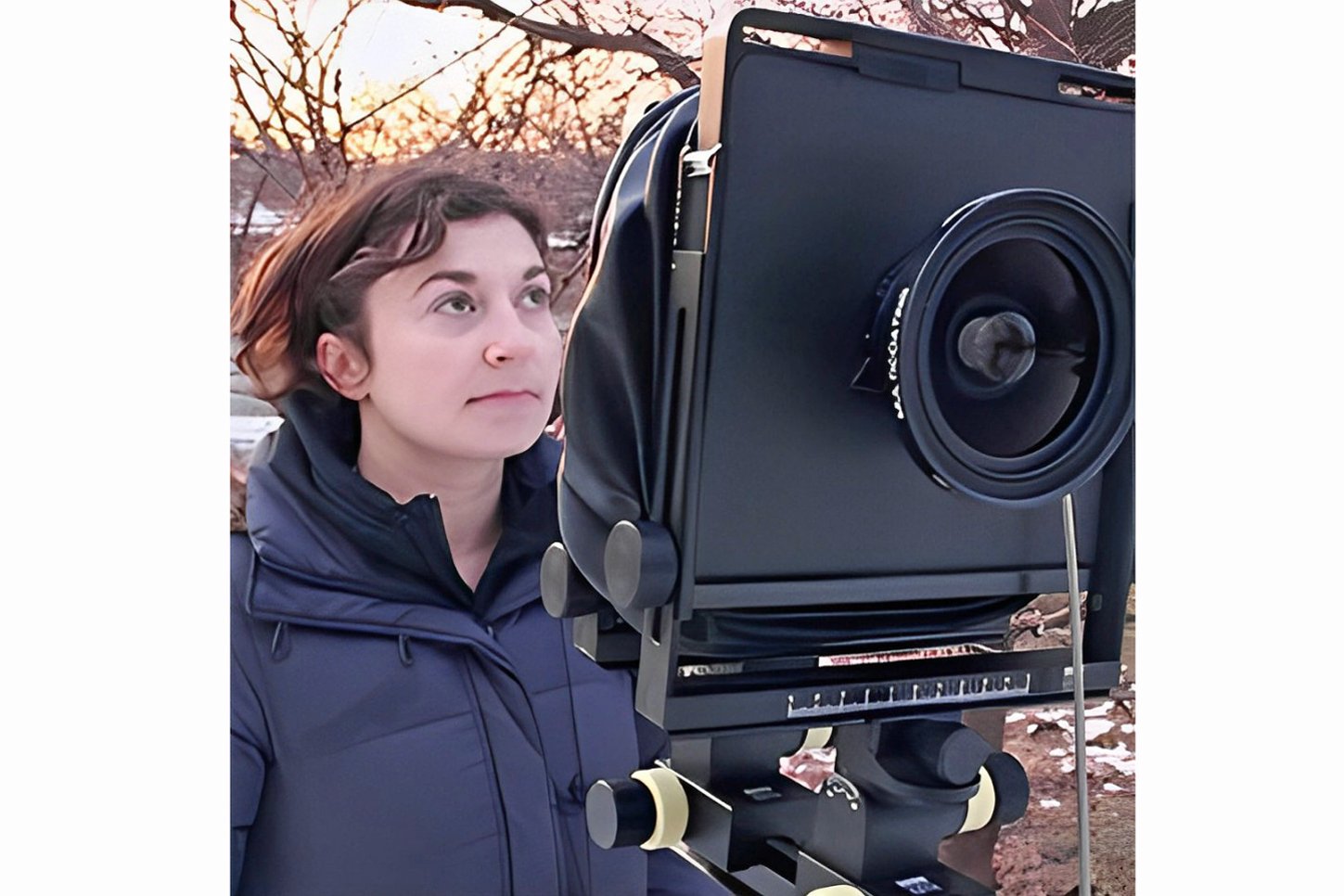The image, likely an altered photograph with soft muted colors, depicts a fair-skinned Caucasian woman with short, slightly curly brown hair standing outdoors, possibly in winter as indicated by patches of snow on the ground. She is located on the left side of the photograph, wearing a dark blue, puffy hooded jacket. Her eyes are directed upwards towards the sky, and she appears to be engaging with a large, vintage camera situated to her right. The camera, which seems to be an 8x10 model with bellows and a substantial lens, stands on a tripod and features several knobs and a dark hood on its back. The background shows bare tree branches and a sky with a yellowish hue, suggesting sunrise or sunset. The overall scene gives the impression that it might be digitally enhanced or created by AI, given the sharp focus on certain elements and the artistic quality of the image.